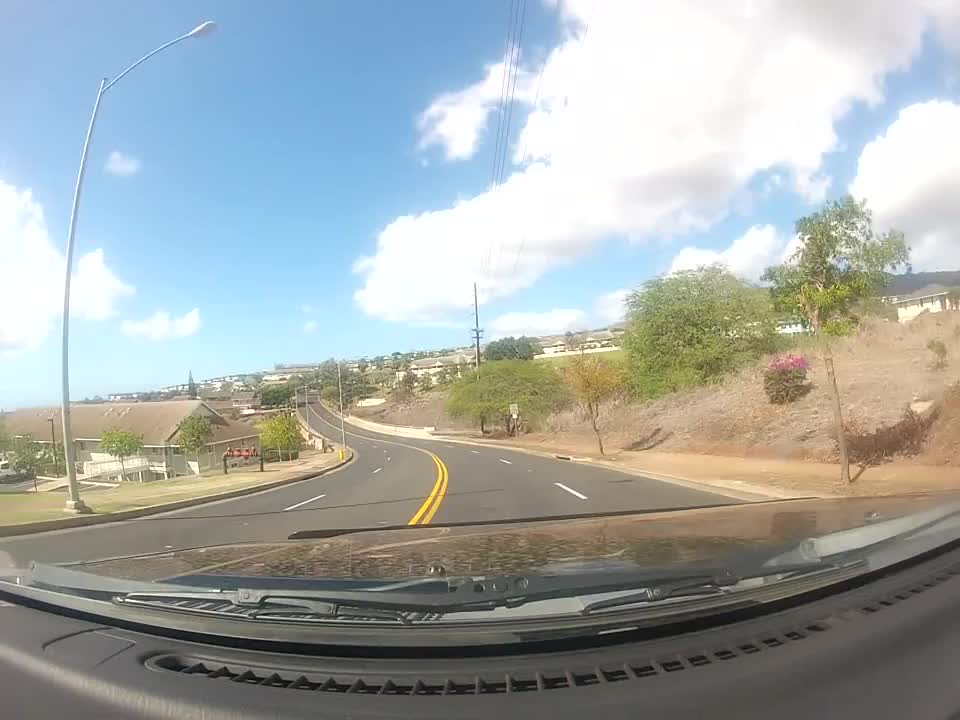A photograph captures the view from the interior of a vehicle, looking out through a reflective black dashboard. The windshield wipers are visible, framing a serene scene ahead. The clear windshield reveals a bright blue sky scattered with a few clouds, setting a picturesque backdrop. The vehicle is navigating a gently curving four-lane road, completely devoid of other traffic, allowing for an undisturbed journey.

Flanking the road, freshly landscaped areas suggest a newer residential development. Young, recently planted trees line the path, complemented by tall street lights and light posts on the left side. The right side showcases small trees interspersed with beds of green and purple flowers, adding vibrant splashes of color to the scene. Brown patches of grass hint at a transitional season or recently completed planting. The entire landscape beautifully reflects off the glossy black dashboard, enhancing the peaceful, newly developed surroundings.